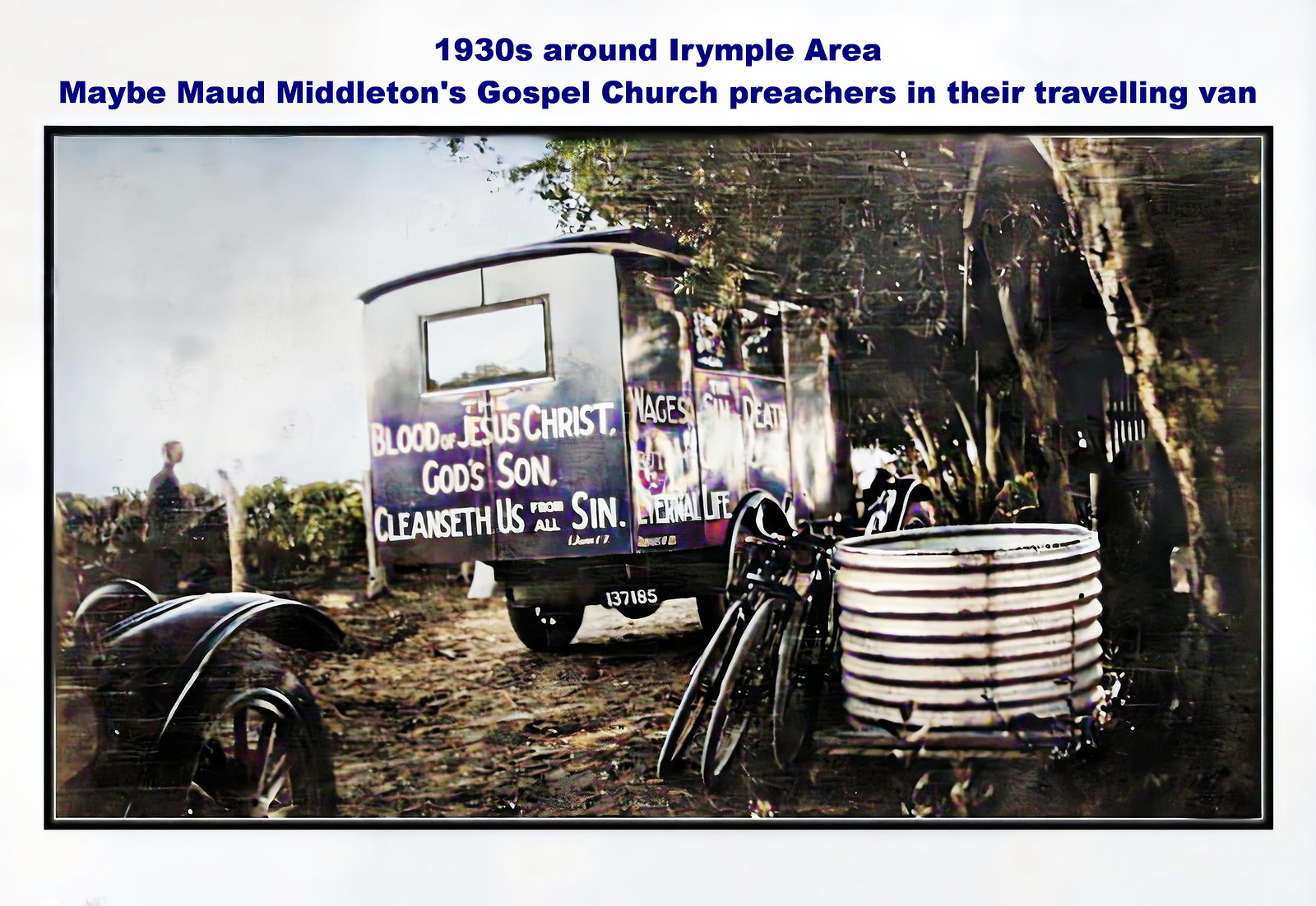The colorized vintage photo, circa 1930s, labeled "1930s around Irnpool area, maybe Maud Middleton's Gospel Church preachers in their traveling van," depicts a dirt area with a large, old-fashioned traveling van at its center. The van, which features text reading, "The blood of Jesus Christ, God's Son, cleanser for us for all sin," on the back and "wages eternal life" on the side, is parked near a small storage trailer amidst a setting with several trees. A black-bordered image displays evident marks and scratches, adding to its historical texture. Surrounding the van on the dirt road are three bicycles leaning against a cylinder tank and the front wheel of a car visible in the bottom left corner, highlighting a pastoral scene typical of rural gospel missions of the era.